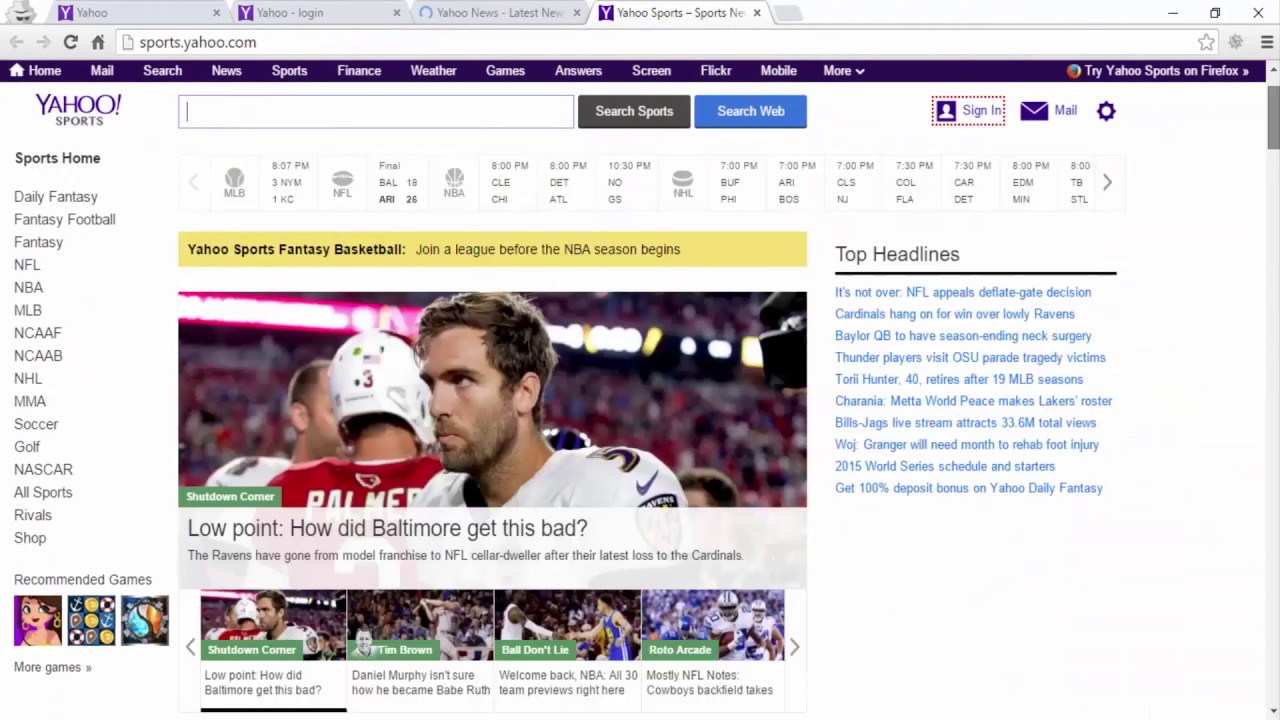**Caption: Screenshot of Yahoo Sports Web Page**

This image is a detailed view of the web page sports.yahoo.com, displayed in a web browser. The interface showcases various sections and navigational options. At the top of the screen, a navigation bar includes links for "Home", "Mail", "Search", "News", "Sports", "Finance", and "Weather". Additional options such as "Games", "Flickr", "Mobile", and "More" are also available. To the right, a banner prompts users to "Try Yahoo Sports on Firefox".

Beneath this, the main content area features the Yahoo Sports logo adjacent to a "Search Sports" box, with a link to "Search the Web" beside it. Sign-in options for a Yahoo account and email, along with a settings icon, are visible as well.

The central headline reads, "Low Point: How Did Baltimore Get This Bad?", with an image of the Baltimore Ravens. Below this, a subheading explains, "The Ravens have gone from model franchise to NFL cellar-dweller after their latest loss to the Cardinals." Beneath the main article, there are four tiles with clickable links to videos:

1. "Shutdown Corner: Low Point - How Did Baltimore Get This Bad?"
2. "Tim Brown: Daniel Murphy Isn't Sure How He Became Babe Ruth"
3. "Ball Don't Lie: Welcome Back NBA - All 30 Team Previews Right Here"
4. "Roto Arcade: Mostly NFL Notes, Cowboys' Backfield Takes"

On the far right of the screen is a section titled "Top Headlines", with blue clickable links leading to various articles and web pages:

- "It's Not Over: NFL Appeals Deflate Gate Decision"
- "Cardinals Hang on for Win Over Lowly Ravens"
- "Baylor QB to Have Season-Ending Neck Surgery"
- "Thunder Player Visits OSU Parade Tragedy Victims"
- "Torii Hunter Retires at 40 After 19 MLB Seasons"
- "Charania: Metta World Peace Makes Lakers Roster"
- "Bills-Jags Livestream Attracts 33.6 Million Total Views"
- "W.O.J.: Granger Would Need Month to Rehab Foot Injury"
- "2015 World Series Schedule and Starters"
- "Get 100% Deposit Bonus on Yahoo Daily Fantasy"

This comprehensive layout of Yahoo Sports provides a blend of news, features, and interactive content for sports enthusiasts.